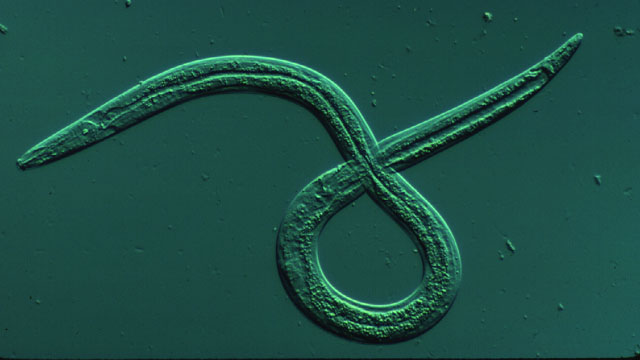This image, captured through a microscope, presents a detailed view of a long, worm-like parasite rendered in various shades of green. The background is uniformly dark green, highlighting the translucent nature of the parasite, which appears almost stained for visibility. The worm, resembling a snake or an earthworm, features a distinctive structure with a central tract likely representing its digestive system. The head, situated in the mid-left section of the image, appears slightly pointy and could be mistaken for having an eye, though this is likely an artifact. The parasite loops and curls around itself, with the tail pointing towards the upper right corner. Despite some minor debris and bubbles on the slide, the focus remains on the intricacies of the parasite’s texture and internal structures, providing a comprehensive demonstration of microscopic photography.